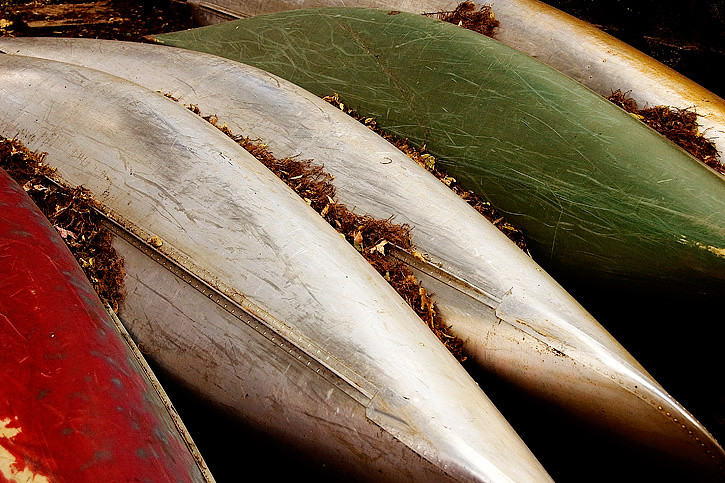The photo depicts five well-worn canoes, aligned side-by-side on a dirt ground, suggesting the end of a season, possibly at a summer camp. The canoes display significant wear and tear; each with numerous scratches and marks, indicative of extensive use. From left to right, the canoes are colored as follows: red, silver, silver, green, and a combination of gold and silver. They are covered with scattered leaves and spruce debris, particularly accumulating in the gaps where the canoes touch each other. The ground is free of grass or rocks, just plain brown dirt. In the background, there's a hint of a wooden platform, and the scene appears to be captured at dusk, as there is a low light atmosphere suggesting the sun is setting.